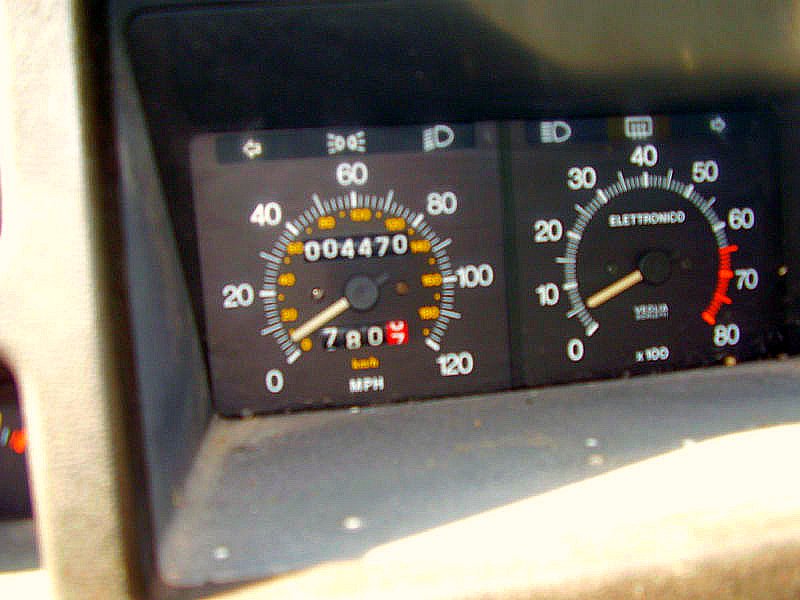A detailed photograph captures the dashboard of a car, focusing on the instrument cluster. The central display shows the odometer reading at 4,470 miles. The speedometer, prominently displayed, registers the speed in miles per hour. Adjacent to the odometer, the tripometer marks 780.6 miles, nearing the 7-tenths mark. Above the speedometer, various indicator lights are visible, including those for headlights, turn signals, and engine status. The engine temperature gauge is prominently at zone 5. Additional control lights, presumably for another set of headlights and turn signals, round out the array of indicators. The photo intricately details the dashboard's instrumentation, providing a comprehensive view of the vehicle's current status.